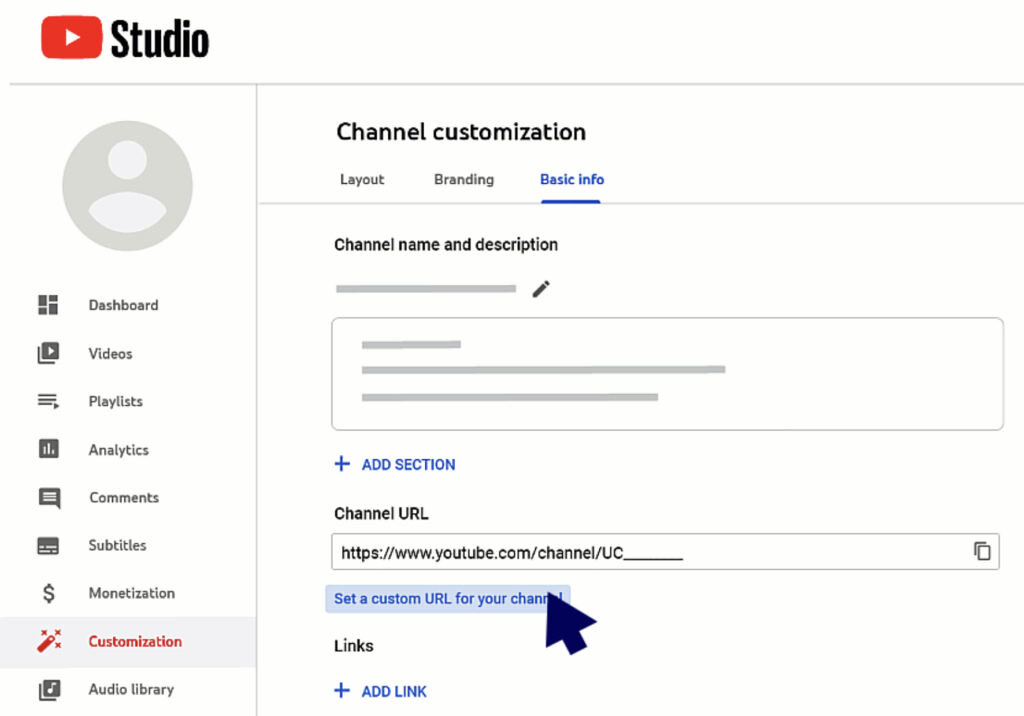The image depicts the YouTube Studio layout. In the top-left corner, the YouTube play button symbol is prominently displayed next to the word "Studio" in black font. Below, there is a circular gray icon resembling a person, consisting of a larger circle with a half-circle underneath.

Under this icon, a vertical menu lists various categories, each accompanied by a distinctive icon:
- **Dashboard:** Icon with several small squares and rectangles.
- **Videos:** Play button with two squares stacked.
- **Playlists:** Lines with a sideways play button.
- **Analytics:** Bar graph icon.
- **Comments:** Speech bubble with lines indicating text.
- **Subtitles:** Black square with white lines.
- **Monetization:** Dollar sign.
- **Customization:** Magic wand with sparkles (this category is currently selected, highlighted in red).
- **Audio Library:** Two gray squares with a musical note.

In the middle section of the image, "Channel customization" is prominently displayed. Below this header, three tabs are listed: "Layout," "Branding," and "Basic info," with "Basic info" selected and highlighted in blue.

Under the "Basic info" tab, the section labeled "Channel name and description" is shown, with placeholder lines indicating where text can be entered, and a small pencil icon for editing. Beneath this, a blue “+ Add Section” button is visible.

Further down, a section titled "Channel URL" is presented. The text box contains a placeholder URL that reads "https://www.youtube.com/channel/UC______." An option to set a custom URL for the channel is also displayed, and a large arrow hovers over this custom URL section.